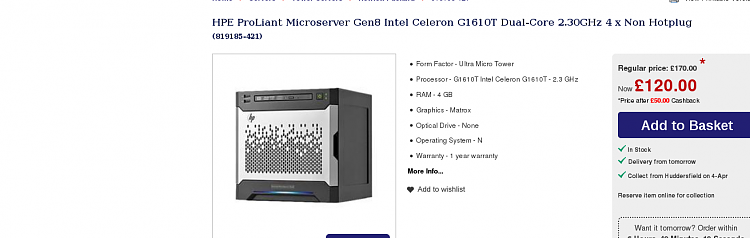The image depicts a product page for the HPE ProLiant MicroServer Gen8, featuring an Intel Celeron 1610T Dual Core 2.3 GHz processor. The product itself is shown prominently on the left-hand side, resembling a box with a unique front panel design that evokes the iconic Matrix rain pattern, albeit in static black and white. This panel stands out against the predominantly black exterior of the device. To the right of the product image, key specifications are listed, detailing the device's form factor, processor, RAM, graphics, and optical drive. Adjacent to these specifications, set against a light blue background, are the pricing information and options to add the item to the basket, facilitating a seamless purchasing process.